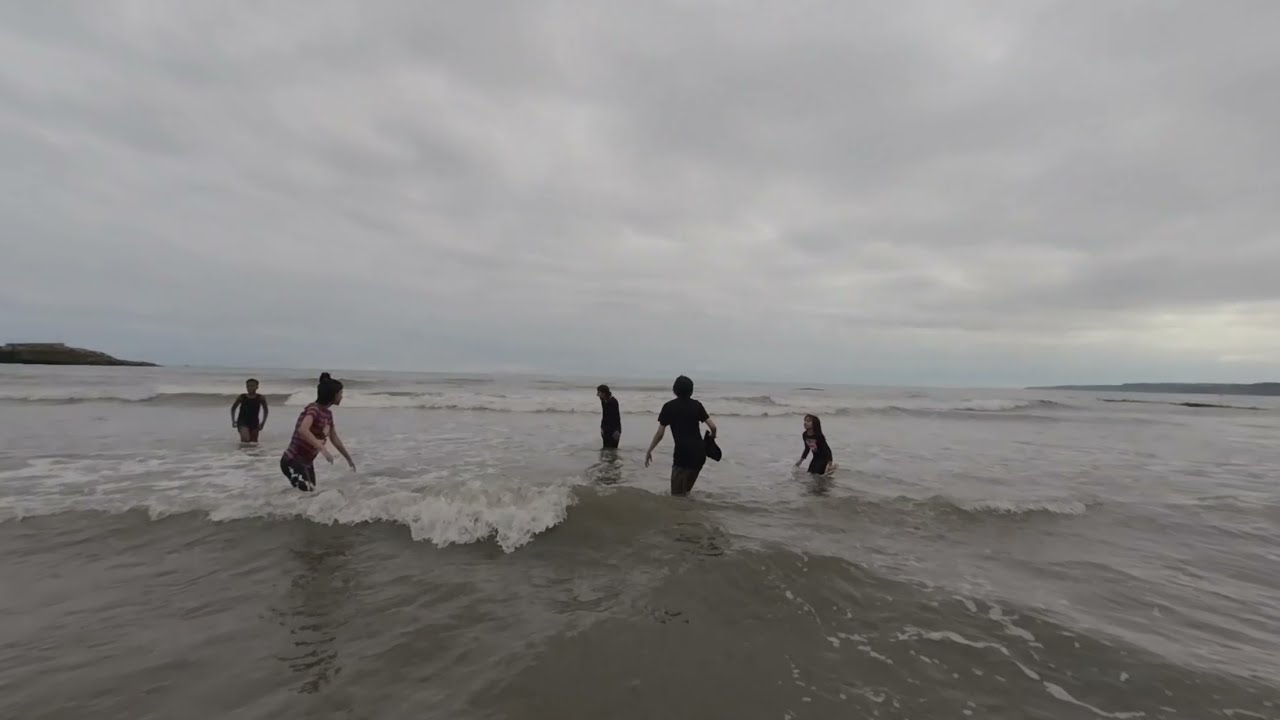In a striking image of an overcast beach scene, five people stand in knee-deep, chilly ocean waters under a cloudy sky that shifts to a darker hue towards the right. The group, dressed in a variety of body suits and long-sleeved tops with one individual sporting a red or rose-colored shirt, appears to be frolicking and interacting with each other. Waves roll gently in both the background and foreground, indicating it might be high tide. On both the far left and right, landmasses are faintly visible, suggesting the setting could be a bay area connected to the open sea. The water itself is a grayish color, adding to the cool, somber atmosphere of this early morning or sunset scene.